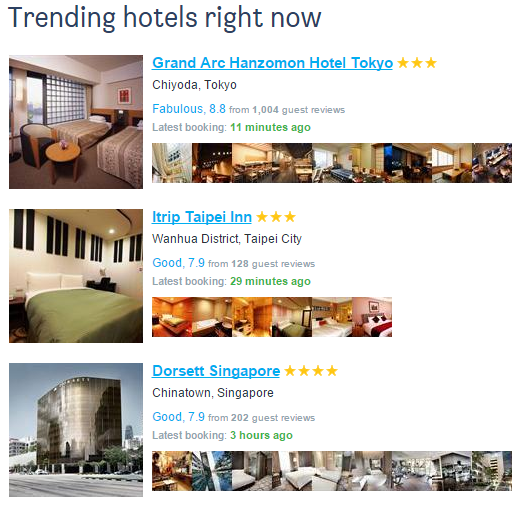**Trending Hotels Right Now**

1. **The Grand Ark Hansaman Hotel**, Chiyoda, Tokyo - *Fabulous* (8.8 from 1,004 guest reviews)  
   - ⭐⭐⭐
   - Latest booking: 11 minutes ago (in green font)
   - Description: The listing showcases an inviting room featuring two beds, a small table, and a chair. There are smaller images displaying various amenities and interiors of the hotel.

2. **iTrip Taipei Inn**, Wenhua District, Taipei City - *Good* (7.9 from 128 guest reviews)  
   - ⭐⭐⭐
   - Latest booking: 28 minutes ago
   - Description: The room boasts white walls, black curtains, a green bedspread, and two white pillows. The advertisement includes smaller images that highlight the hotel's interior features.

3. **Dorset**, Chinatown, Singapore - *Good* (7.9 from 202 guest reviews)  
   - ⭐⭐⭐⭐
   - Latest booking: 3 hours ago
   - Description: The exterior shot reveals a sleek hotel with reflective black windows. Similar to the other listings, a reel of images provides a closer look at the hotel's amenities and interior spaces.